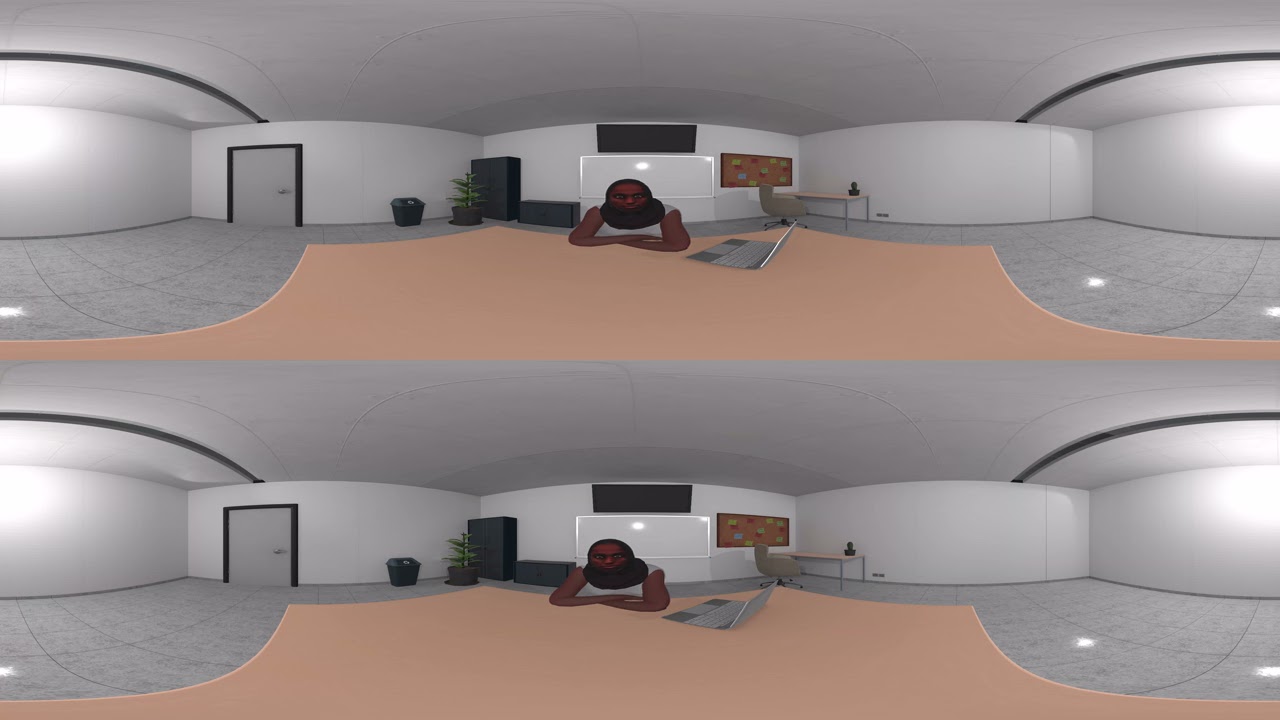The image is a horizontally stretched, computer-generated panoramic scene duplicated across the horizontal axis, resulting in the same image appearing on the top and bottom halves. It depicts a spacious conference room with consistent white walls and ceiling, complemented by gray tiled flooring. In the central focus is an African-American individual, possibly male, distinguishable by a black beard and seated at a large beige table with arms folded and a laptop in front. The background, from left to right, includes a gray door with black outlining, a plant, black furniture or cabinets, and a whiteboard positioned above a bulletin board. Additional details include a trash can near the cabinets, and in the far right, another desk and chair. The room's minimalist design is underscored by the uncluttered walls and simple furnishings.